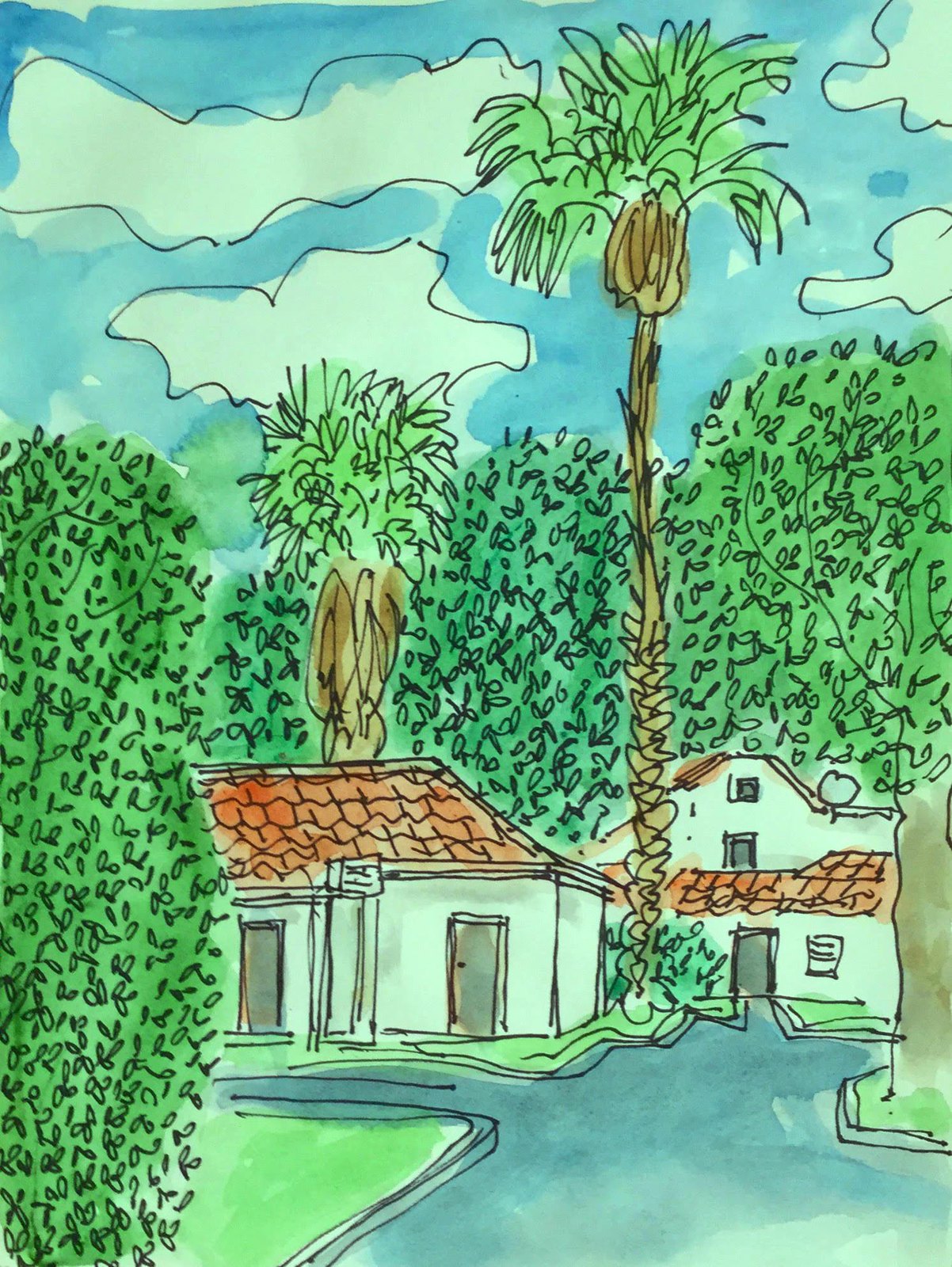This captivating watercolor painting depicts a charming house nestled in a tropical paradise. The residence features a striking orange terracotta tile roof that contrasts beautifully with its light tan walls, exuding a warm and inviting ambiance. Encircling the house is an abundance of lush, dense deciduous trees, their foliage displaying a vibrant spectrum of greens ranging from vivid grass to deep emerald hues. This verdant canopy creates a serene and picturesque setting.

Prominent in the scene are two majestic palm trees. The first, an impressively tall specimen, stands proudly to the right of the house, its fronds waving gently above the roofline. The second palm, slightly shorter and more discreet, peeks from behind the house to the left, adding to the tropical aesthetic.

In the foreground, a dark blue road winds in front of the house, suggesting accessibility and connection. The road appears to lead not only to this residence but extends towards the neighboring house, hinting at a close-knit community nestled in this lush haven. The tree trunks, rendered in a rich walnut brown, provide a grounding contrast to the otherwise green-dominated landscape, enhancing the overall depth and realism of the scene.

This detailed watercolor captures the essence of tropical living, with its harmonious blend of natural beauty and serene architecture.